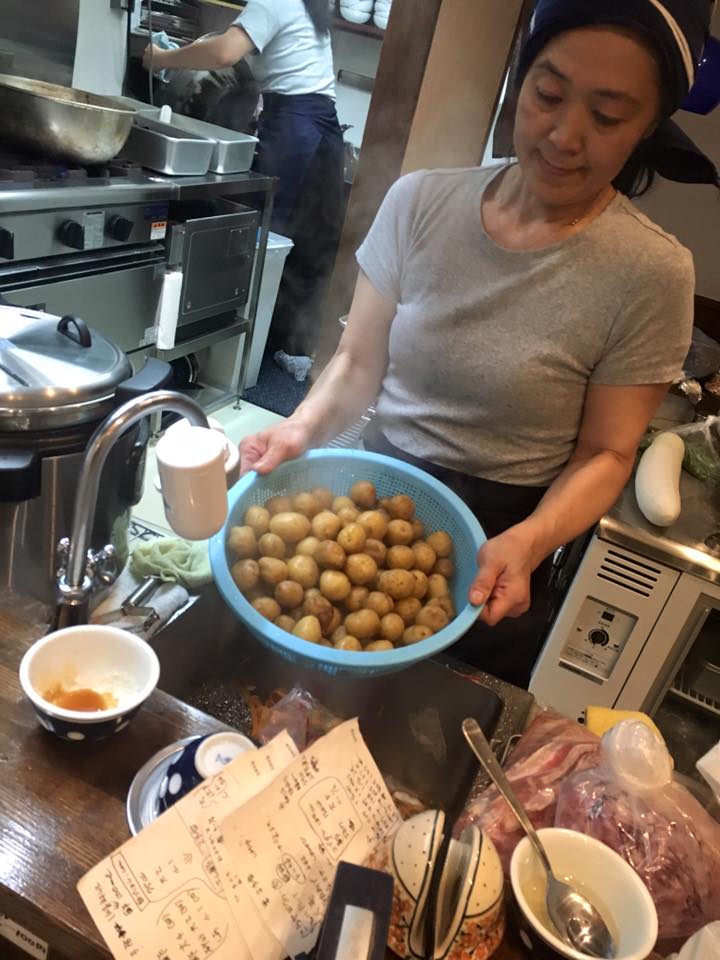In this vertically oriented, realistic photograph, we see an Asian woman, possibly in her 30s, standing in a bustling kitchen that appears to be part of a restaurant or a take-out venue. She’s dressed in a short-sleeved gray t-shirt, blue pants, and a blue hat or headband. The woman is holding a large blue bowl filled with small yellow potatoes, rinsing them under the sink on a stainless steel work surface that features a wooden counter edge. 

The backdrop reveals a busy kitchen with light beige walls, industrial-sized stainless steel appliances including a large stove, an oven, and numerous pans and pots. A couple of white pieces of paper with black writing, likely orders, are scattered around. In the background, another person is engaged in cooking, dressed in a white short-sleeved shirt. The scene is filled with food items and utensils, emphasizing the active and professional nature of this kitchen environment.